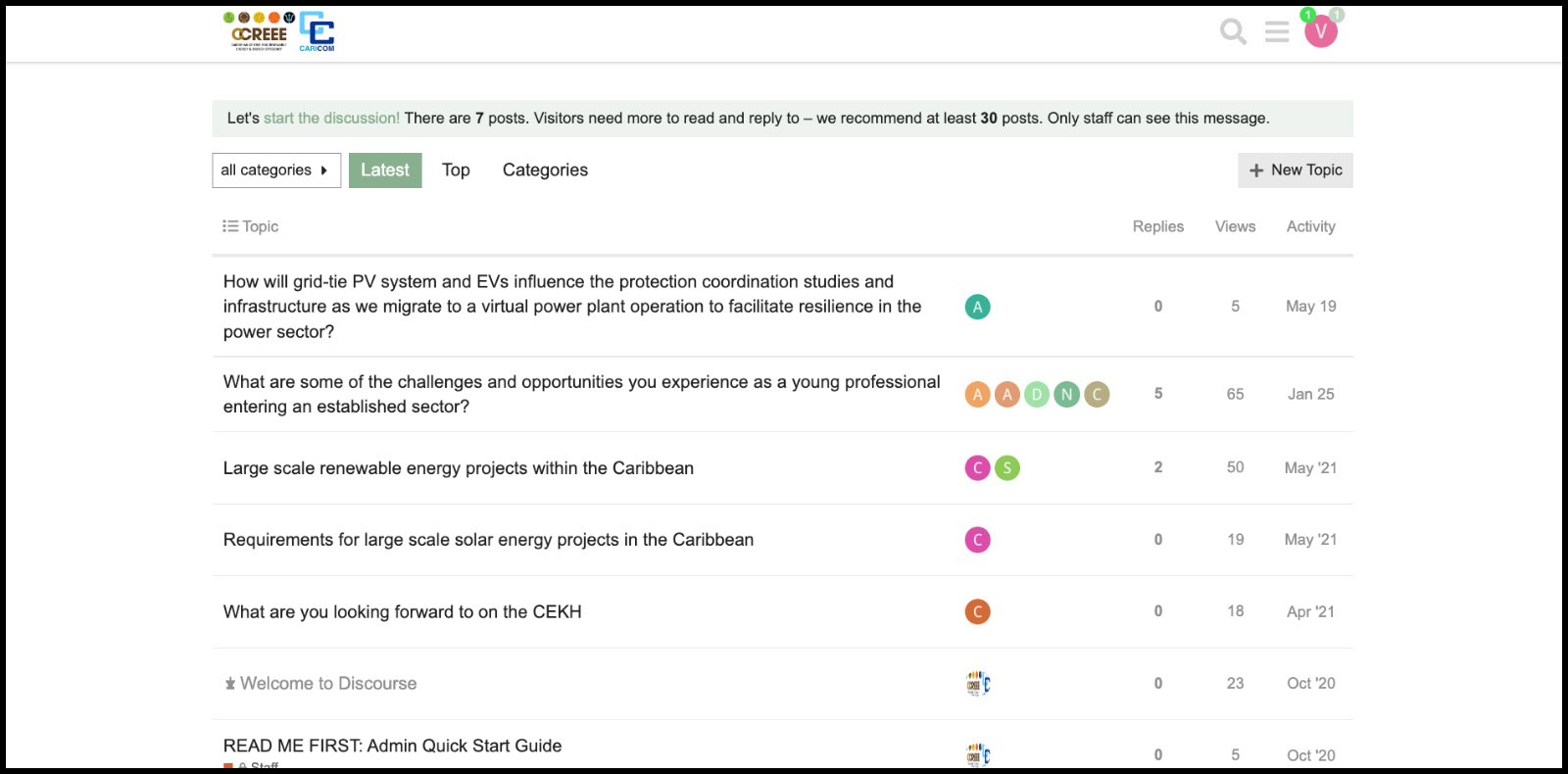This screenshot captures an interface of a web-based discussion forum, possibly named "CREE," although the exact name is unclear due to its small font size. The layout of the application prominently features several user-friendly elements designed to facilitate forum navigation and interaction. At the top of the screen, there are filtering options including "All Categories," "Latest," "Top," and "Categories," allowing users to sort through various discussion threads. 

The main section of the screen displays a list of topics that have been posted by users. Each topic is clickable, directing users to view individual discussions in detail. Adjacent to each topic, there are columns that neatly show key metrics for each discussion: the number of replies, the number of views, and the timestamp of the latest activity. This structured design aids users in quickly gauging the popularity and recency of each discussion thread.